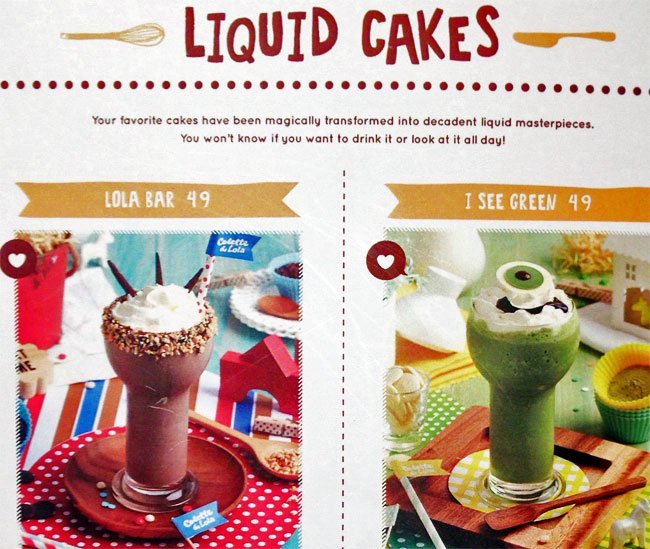The image is a digital ad set against a light gray background, showcasing two types of liquid cakes positioned side by side. At the top of the image, the title "Liquid Cakes" is prominently displayed in large red letters. Just below this, a red dotted line runs horizontally across the width of the image, separating the title from the rest of the content. Below the dotted line, the slogan reads: "Your favorite cakes have been magically transformed into decadent liquid masterpieces. You won't know if you want to drink it or look at it all day."

On the left side, above the image of a liquid cake, it says "Lola Bar 49." This liquid cake is presented in a sundae glass, with a mixture resembling a strawberry swirl. The glass is beautifully adorned with whipped cream on top and its rim is coated in chocolate syrup and nuts. The dessert is artfully arranged on a red plate. 

On the right side, above the second image, it says "I See Green 49." This liquid cake also comes in a similar glass, featuring a vibrant green liquid. The top is decorated with whipped cream and a green fondant resembling an eyeball. This dessert is placed on a square, yellow and white plate.

Additional decorative elements include a small red circle with a heart at the top left corner of each photo. The overall presentation emphasizes the unique and enticing visual appeal of these liquid cakes, blending the lines between a delightful treat and an artistic masterpiece.